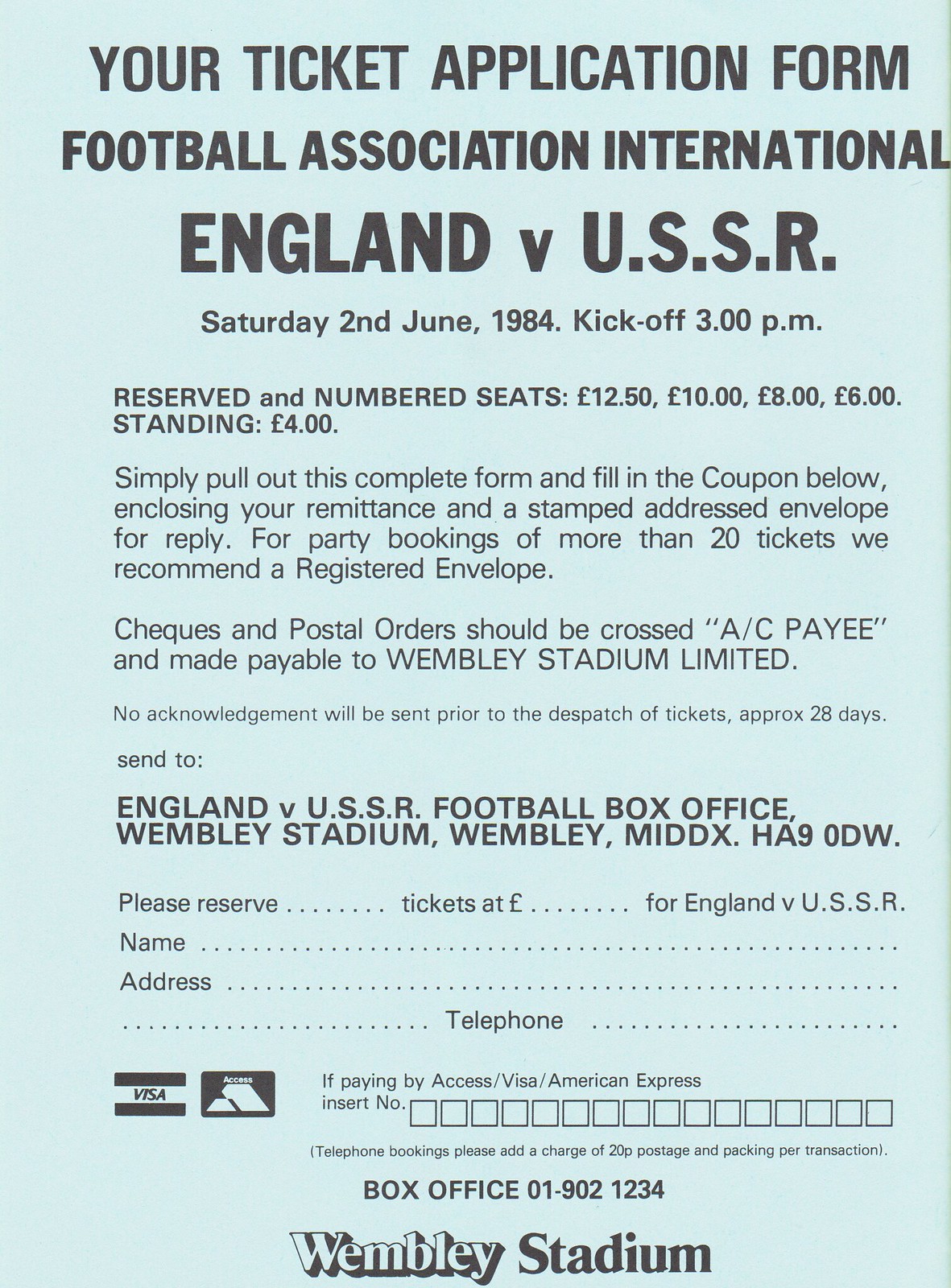The image depicts a light blue paper with black text, serving as a Ticket Application Form for a football match organized by the Football Association International. At the top, it reads "Your Ticket Application Form," followed by "Football Association International" and "England V USSR." The match is scheduled for Saturday, 2nd June 1984, with kickoff at 3 p.m. The form mentions reserved and numbered seats, with ticket prices listed as £12.50, £10, £8, £6 for standing, and £4. It includes instructions to fill out the form at the bottom, which requires personal details such as name, address, phone number, and credit card information. Additional directions mention enclosing remittance and a stamped addressed envelope for reply, with a recommendation for a registered envelope for party bookings of more than 20 tickets. Payments should be made via checks or postal orders to Wembley Stadium Limited. The address for submission is "England v. USSR Football Box Office, Wembley Stadium, Wembley Midwicks, HA9ODW." The form also features Visa and Access logos and reiterates "Wembley Stadium" at the bottom.